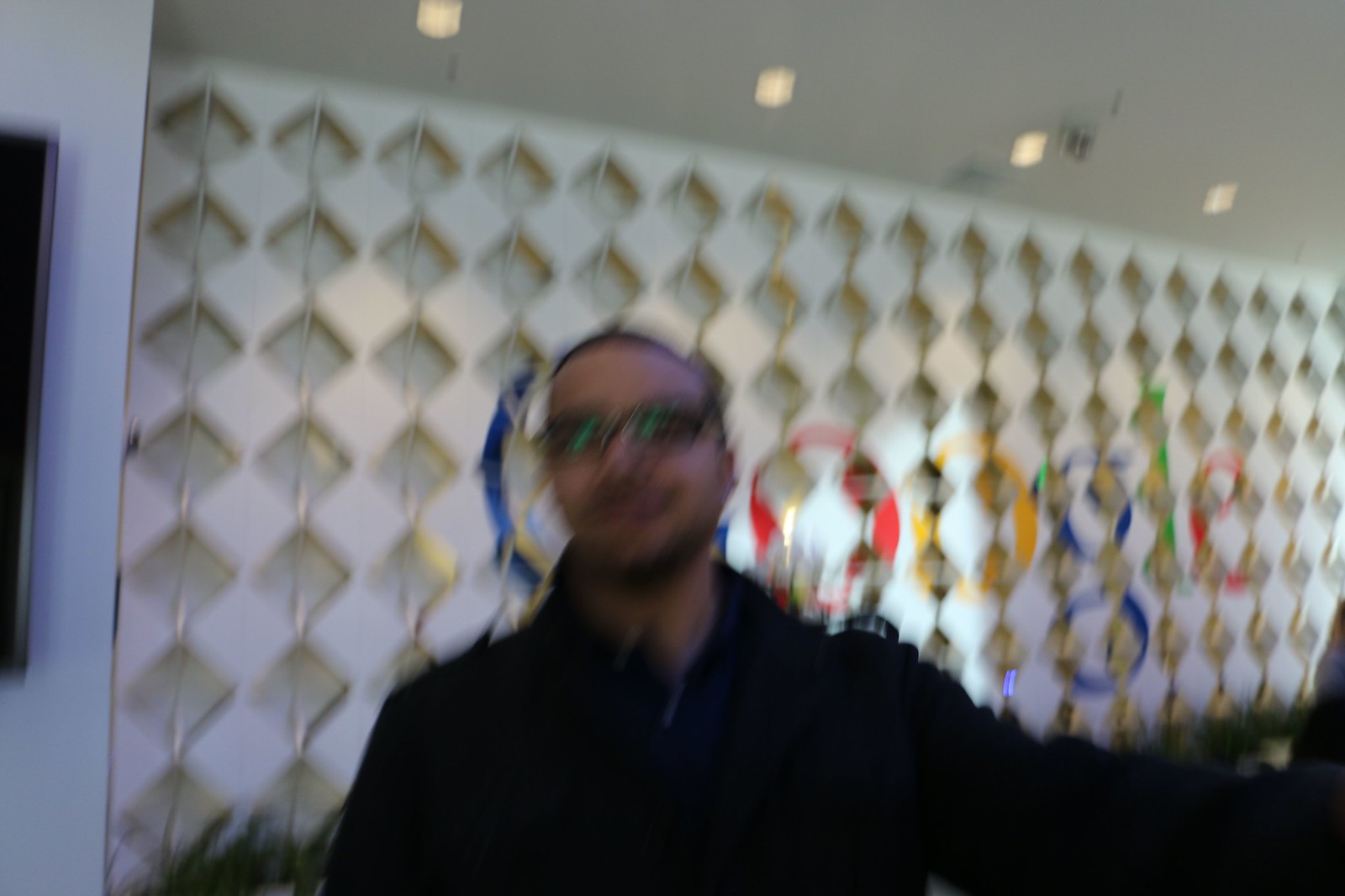In this horizontally shot color photograph, a person appears prominently in the blurry foreground. The individual, possibly male, is dressed in a dark shirt or perhaps a black jacket. They have short hair and exhibit some facial hair, which could be a mustache, beard, or simply a five o'clock shadow. Despite the blur, their smile is discernible, and they are wearing glasses that might be tinted or sunglasses. The background features an ornate wall adorned with numerous diamond-shaped cutouts and illuminated by lights. Positioned on this wall is the iconic Google logo in its signature blue, red, yellow, and green colors, suggesting the setting is within a Google office or a space affiliated with the company.